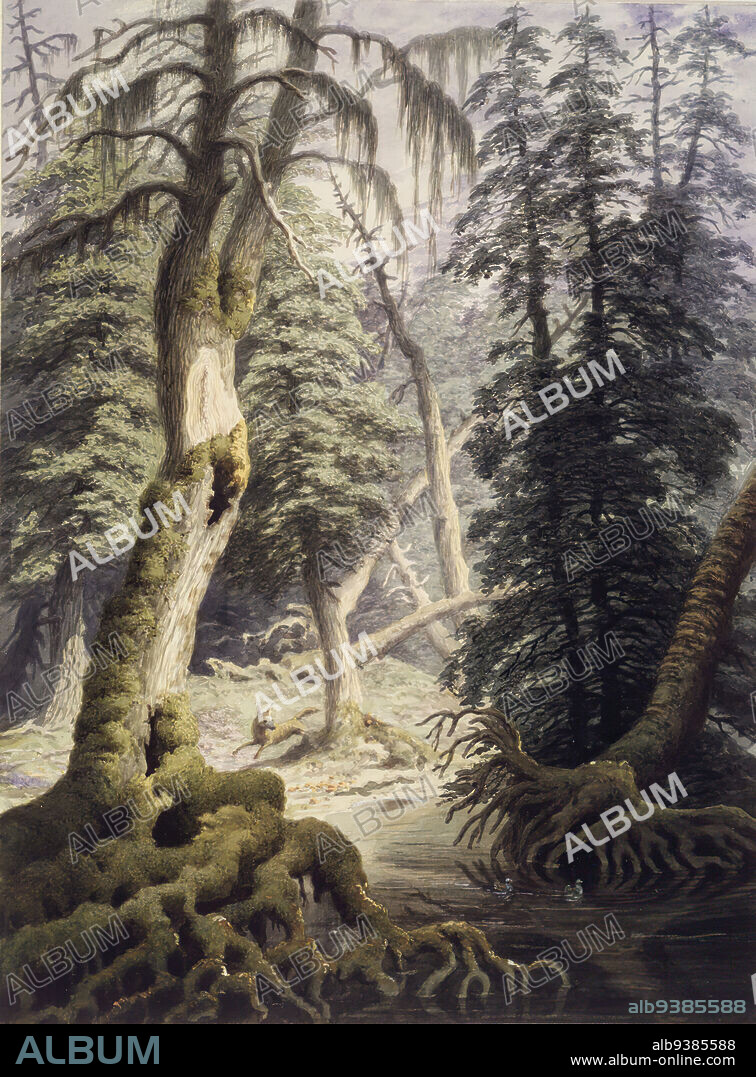The artwork is a detailed and vibrant forest scene rendered in a realistic yet artistic manner, likely a drawing or digital art piece. Dominating the middle ground is a small wolf, running through the forest, which includes a mix of tree species such as pines and possibly oaks. Some trees appear to be uprooted, with expansive roots exposed and covered in moss, while others have Spanish moss draping from their branches. A small stream or river cuts through the scene, with some trees standing in the water. The sun filters through the canopy, casting light in patches across the forest floor. The sky is visible with hazy clouds, suggesting it's daytime. The artwork is heavily watermarked with the word "ALBUM" in various styles of white and clear fonts, and features a numeric code "LB9385588" along with the text "ALBUM" and the website "www.album.com" at the bottom. The repeated watermarks and details attest to its significance as a piece from an album collection.